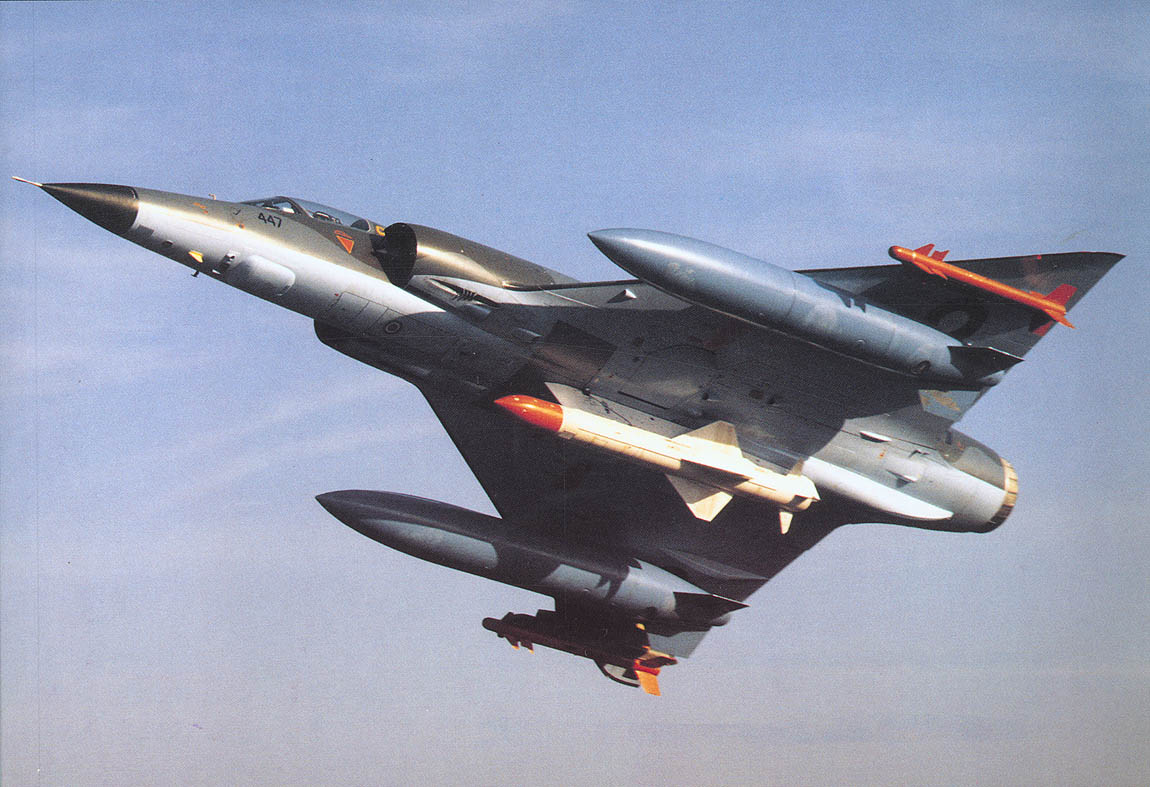The image features a modern fighter jet soaring through a clear, light blue sky adorned only with very faint clouds, illustrating a beautiful day. The perspective is from below, gazing upwards at the aircraft as it heads towards the left of the frame, with its triangular shape accentuated by the black nose tapering back into a silver body. Near the cockpit, the number "463" is visible. The jet is armed with an array of missiles: two gray missiles are mounted on either side, smaller red missiles are positioned further out on the wings, and a white missile with an orange-red tip is centrally located beneath the plane. A subtle shadow of the jet can be seen, enhancing the detail and depth of the image.